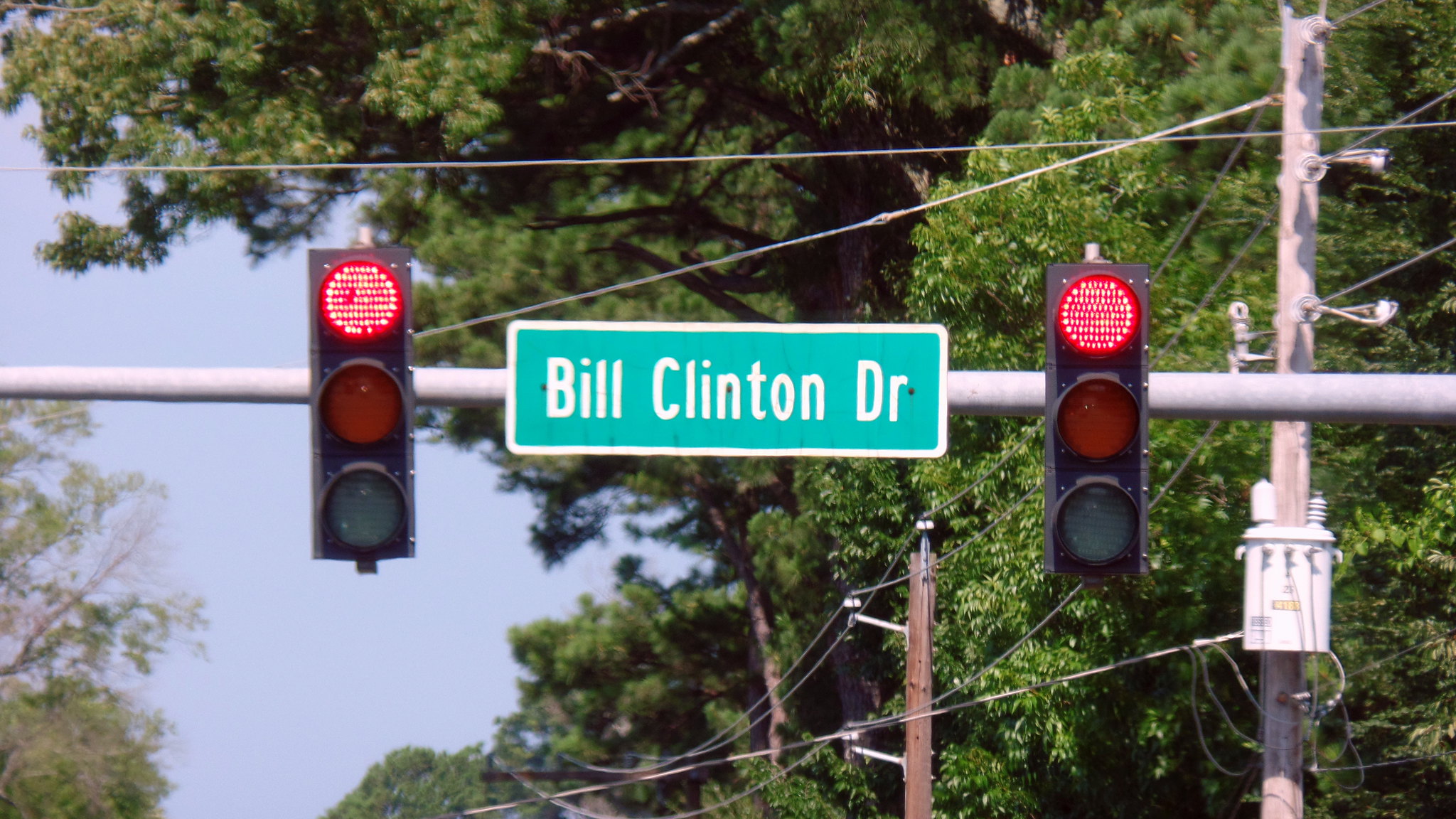In this realistic photograph captured in a suburban area, the central focus is a tall metal pole with a prominent green street sign edged in white, displaying "Bill Clinton Drive" in bold white letters. Flanking the street sign on either side are two traffic lights, both glowing a bright red. Just behind this central feature, a telephone pole stands adorned with a transformer box, from which an intricate web of wires stretches out, connecting to another series of telephone poles that recede into the distance along the street. The backdrop reveals a clear blue sky, indicating it is daytime, with lush green trees filling the scene. The trees are densely grown with vibrant green leaves and interspersed with brown branches, providing a natural canopy. On the right side of the image, numerous trees are visible, while a few trees appear on the left, framing the photograph with their verdant presence.